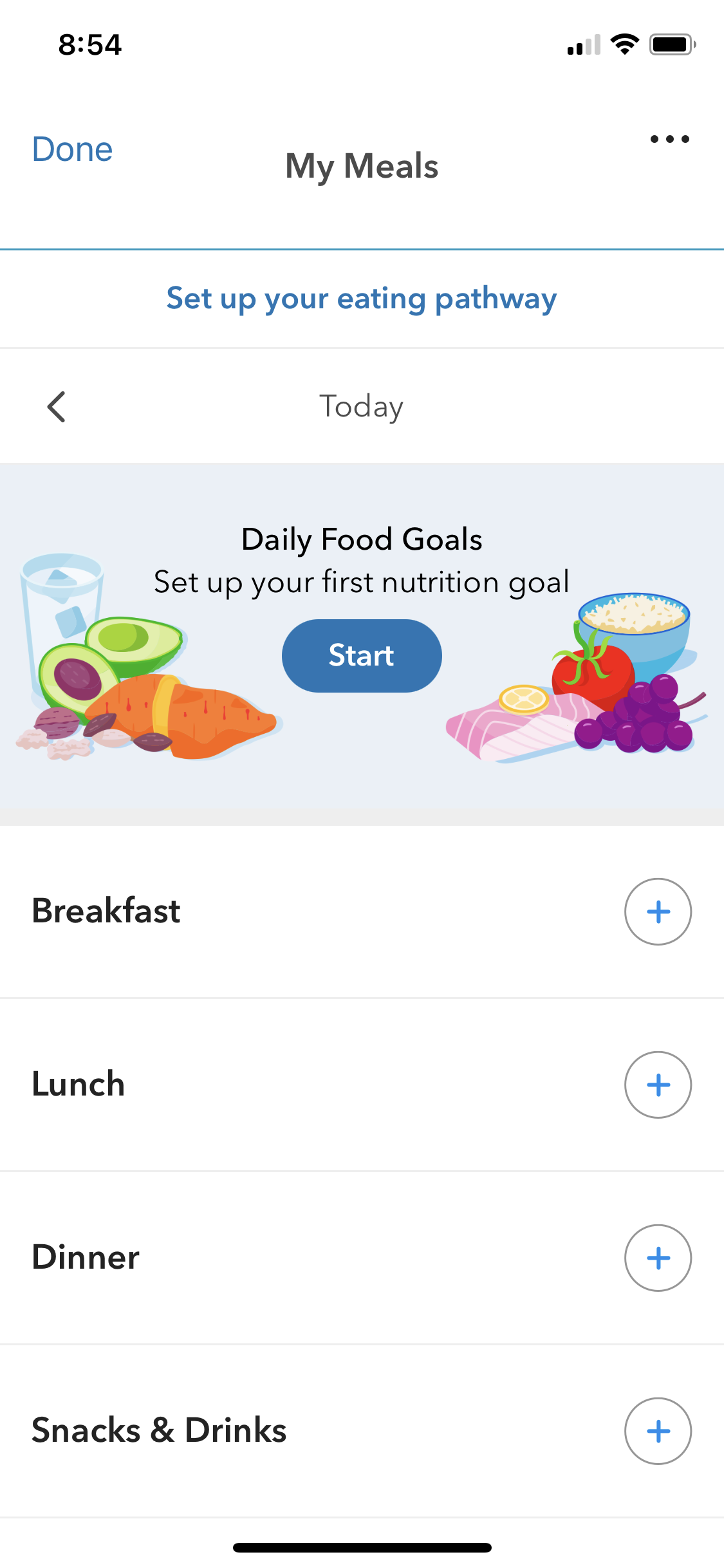This is a screenshot from a mobile application displaying a section titled "My Meals." The interface is predominantly white, with black text providing clear contrast. The main content of the screen includes daily food goals and a prompt encouraging users to set up their work nutrition goal. There's a visually sectioned area showcasing an assortment of healthy food options, including avocados, sweet potatoes, nuts, a glass of water, and a bowl of rice.

The application categories meals into "Breakfast," "Lunch," "Dinner," "Snacks," and "Drinks," each clearly labeled in bold black font. A prominent "Start" button invites users to begin tracking their dietary intake. Additional options, such as setting up an eating pathway, are promoted to help maintain a structured record of meals. 

At the top-right corner, a "Done" button is available for finalizing entries. Indicators at the top of the screen show the user is connected to Wi-Fi and the battery is nearly full. There are also three vertical dots representing further menu options, and a timestamp displaying 8:54.